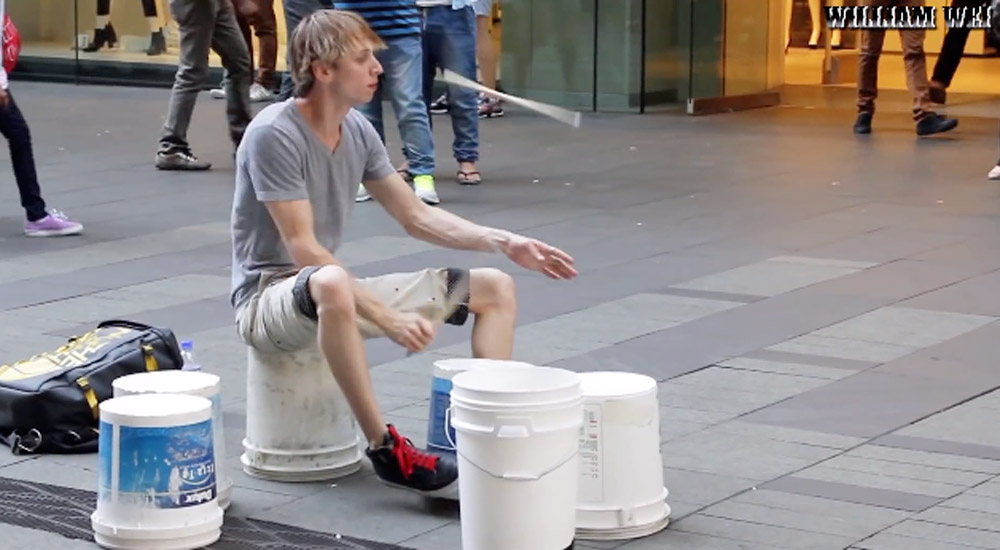In this photograph, a slender Caucasian street performer is captured performing on a bustling city walkway. The performer, clad in a grey t-shirt and khaki shorts, is seated on an upside-down white bucket amidst several other white buckets arranged around him - four turned over and one upright. He wears black sneakers with red laces and has short dirty blonde hair. As part of his dynamic drumming act, one drumstick is seen striking a bucket while the other is skillfully twirled through the air. A black backpack and a water bottle lie on the ground behind him. A backdrop of tiled pavement and what appears to be an entrance to a shopping store hints at the urban setting, while the visible legs and footwear of passersby suggest a busy and well-traversed area. Additionally, in the upper right corner of the image, the word "William" is partially discernible, possibly indicating a nearby store or advertisement.